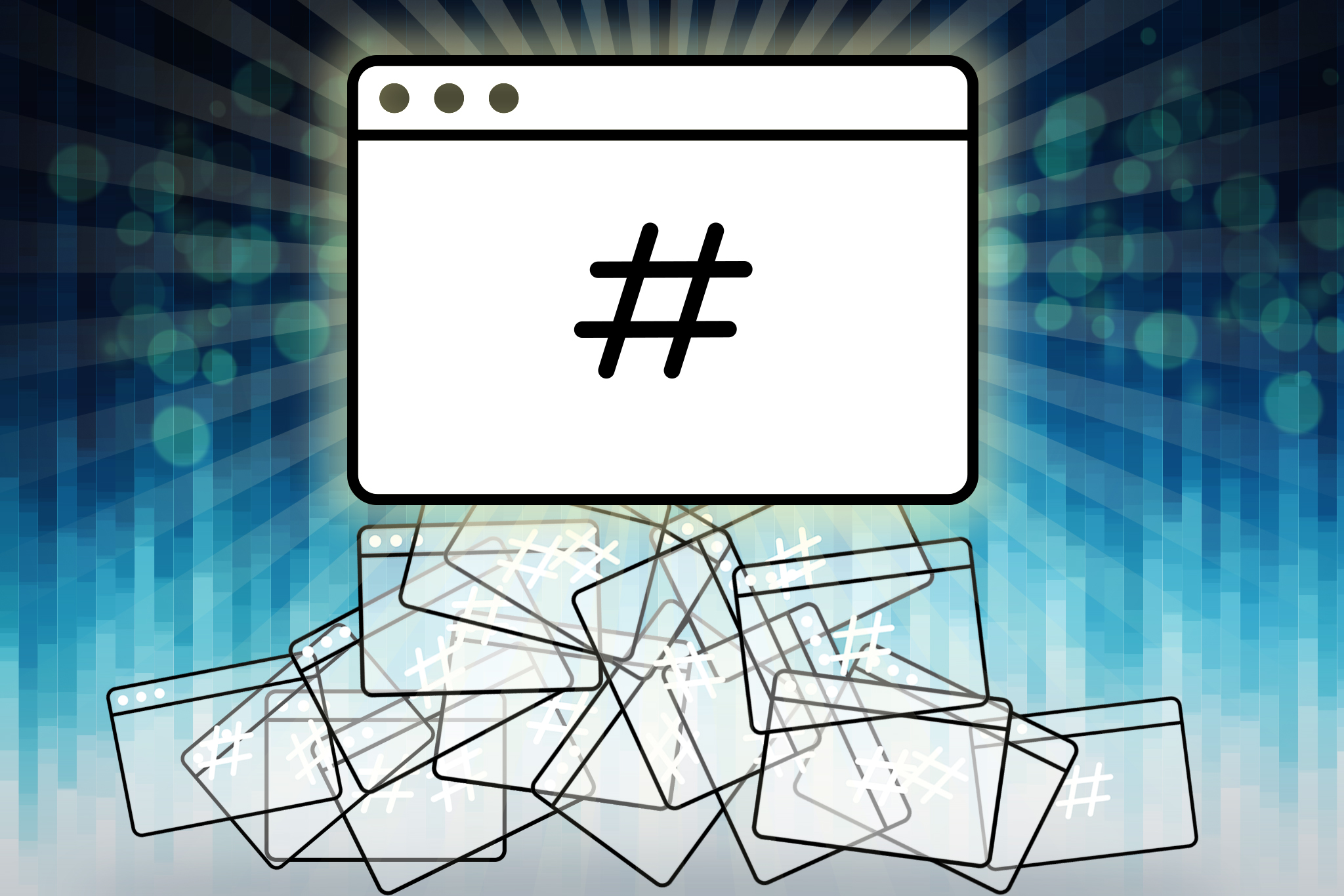The image depicts a digitally generated, horizontally-aligned rectangular interface with a central focus on a browser window. This window, shaded in white and outlined in black, centrally features a prominent black hash symbol (often called a pound sign or octothorpe). The top section of the browser window includes a horizontal line creating a header area with three dark brown buttons on the left side, used for minimizing, closing, or other window functions. Surrounding the main window is a cascade of semi-transparent, rectangular outlines, each mirroring the central window, complete with faint hash symbols. These outlines appear to be stacking or floating towards the image's bottom center. The background transitions from dark blue at the top to lighter blue and finally gray at the bottom, with an overlay of diffused rays emanating from the center. These radiating lines glow in a light gold or white hue, accompanied by small, faint circular dots resembling bubbles or greenish light spots, enhancing the digital and radiant quality of the scene.